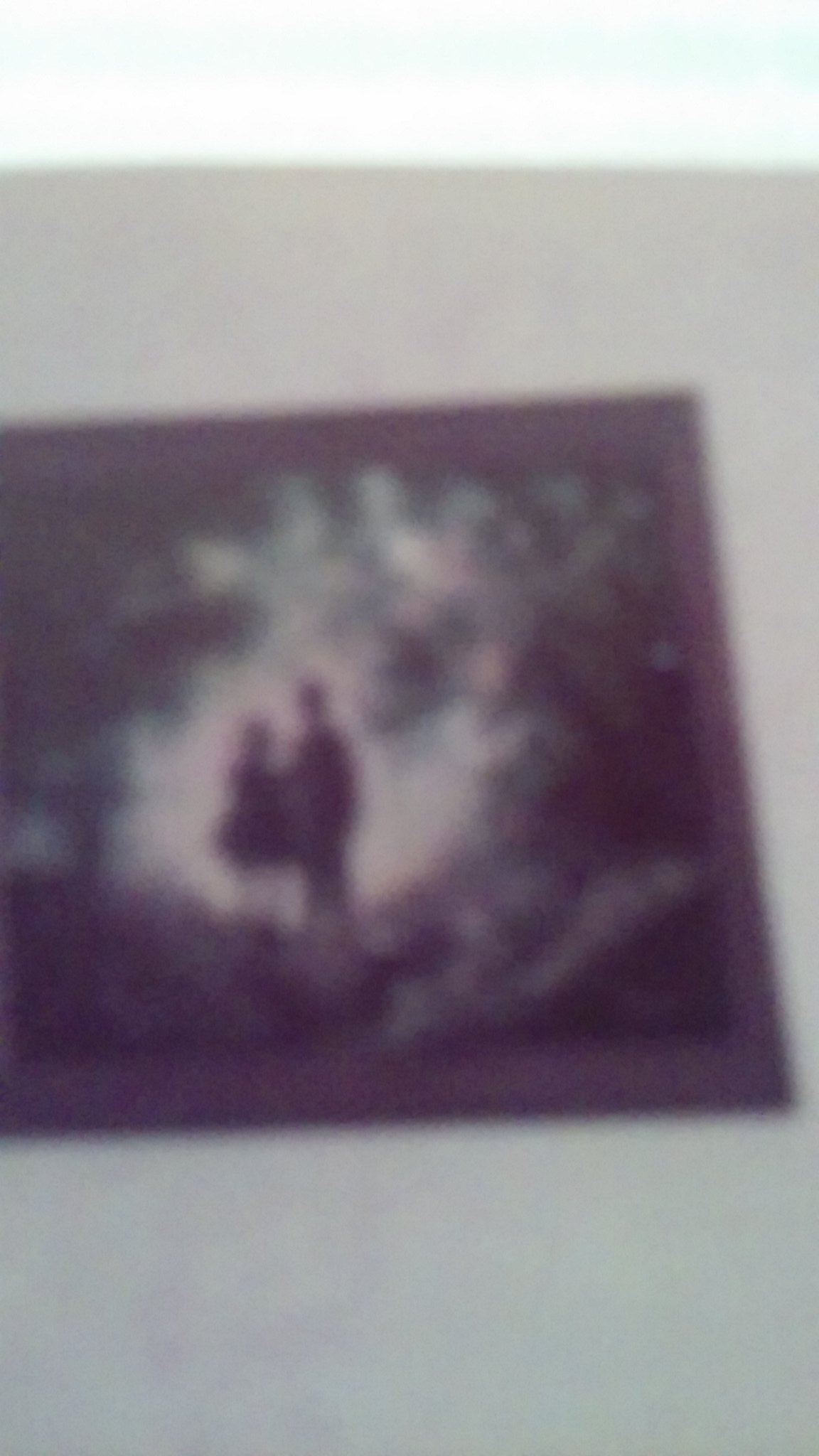This photograph captures a very blurry image of a large square painting in a black wooden frame situated on a light gray wall. The painting itself features an indistinct scene, blurred to the point where only silhouettes are discernible. Central to the painting are two figures, a man and a woman, standing side by side and slightly turned towards each other. The woman, recognizable by her dress, and the man are illuminated by a circle or tunnel of light behind them, casting their forms in stark silhouette. Surrounding this central light, the painting transitions into progressively darker shades of gray and black, contributing to a sense of depth and possibly suggesting a woodland or outdoor setting. The vague hint of green in one corner might indicate foliage or trees. Overall, the indistinct details create an intriguing, almost mysterious atmosphere.